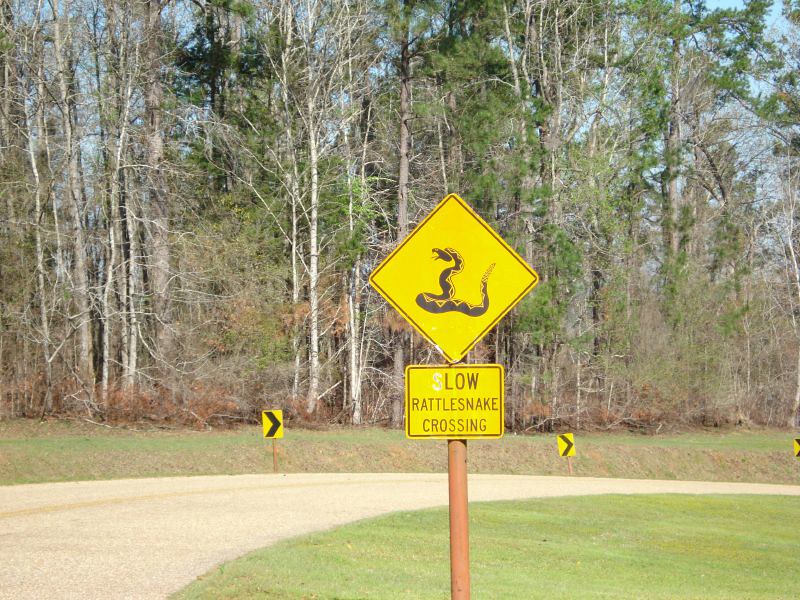In the image, a light brown pole ascends from the bottom, supporting two prominent yellow signs. The lower sign is square with a bright yellow background and bears the cautionary message "Low Rattlesnake Crossing" in bold black text. Above it, a diamond-shaped sign of the same vivid yellow background showcases a striking black and orange rattlesnake illustration. The scene is set in a grassy field that curves gently to the right, juxtaposed against a light gray road that winds to the right as well. Along this road, three distinct yellow square signs with black arrows pointing to the right provide additional guidance. In the background, a sprawling field mixes shades of brown and green, leading up to a line of trees. These trees, adorned sparsely with green leaves amidst mostly gray branches, stand out against the softer, muted hues of the landscape.